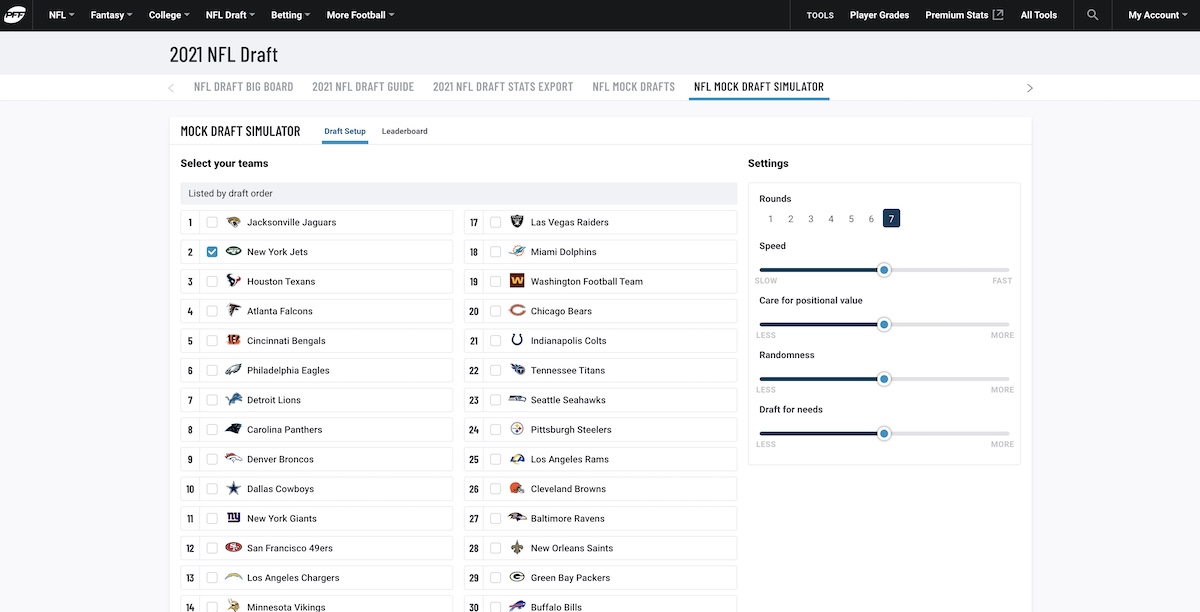An image displaying a webpage with a black header featuring the NFL logo and titles related to fantasy football and the NFL Draft. The main content includes various categories such as the "2021 NFL Draft","NFL Draft Big Board," "2021 NFL Draft Guide," "2021 NFL Draft Stats," and an "Export" function. There are also mock draft tools, with an "NFL Mock Draft Simulator" highlighted in blue and a "Draft Leaderboard." The page background is white, and there is an option to "Select Your Teams and Settings," followed by a list of teams numbered from 1 to 50. A magnifying glass icon is present, suggesting a search function. Comprehensive player grades and premium site content appear to be available.